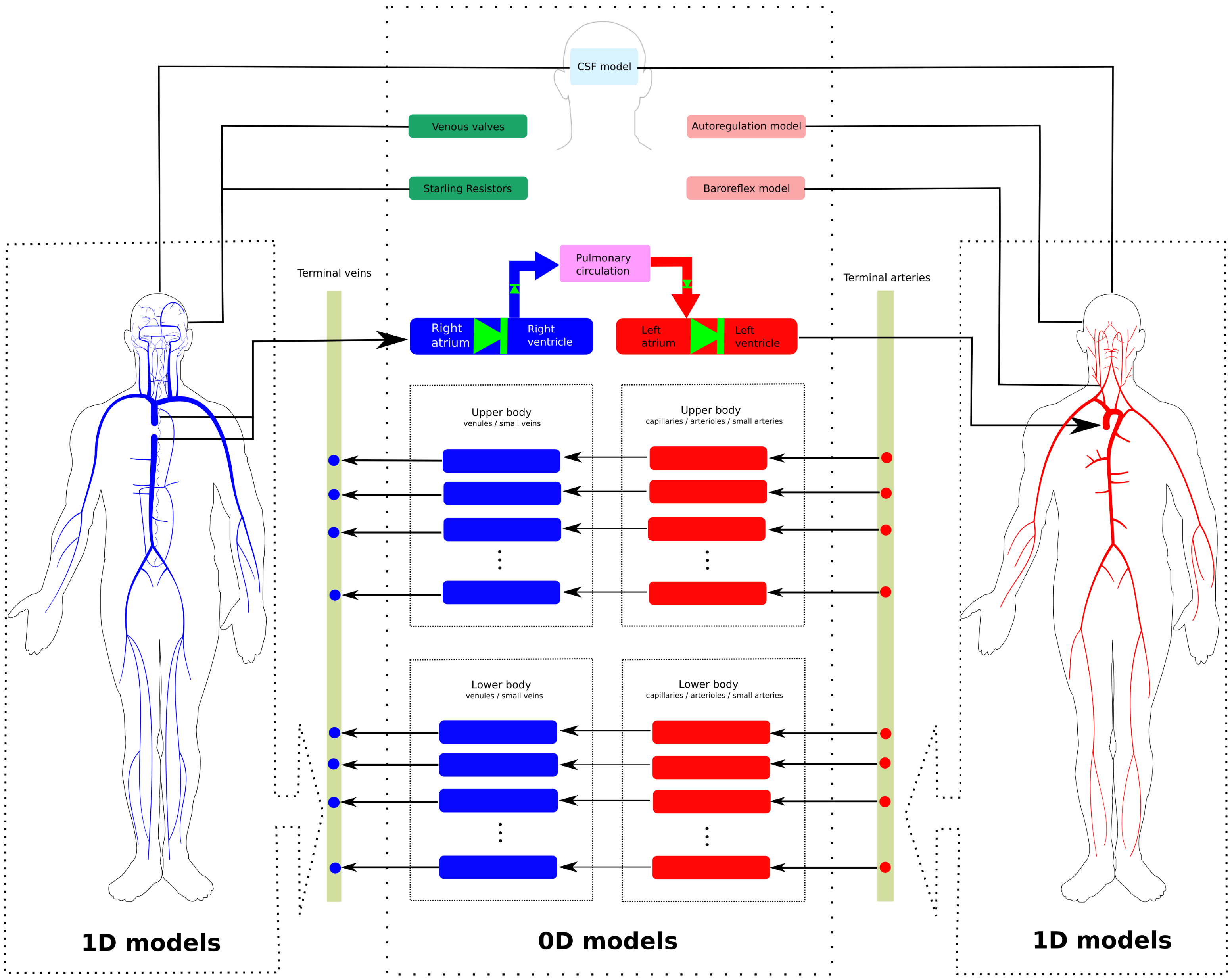The image is a detailed, color-coded textbook diagram illustrating the circulatory system, with an emphasis on pulmonary circulation and blood flow. The diagram consists of two clear human body outlines, one on the left and one on the right. The left side highlights the venous system with blue, representing deoxygenated blood, while the right side features the arterial system in red, showing oxygenated blood. There are numerous lines and arrows pointing to key structures, with annotations that include terms like venous valves, Starling resistors, autoregulation model, and baroreflex model.

Both body outlines are labeled as D1 models, while the center section, noted as OD models, contains detailed explanations and additional annotations. The diagram includes labels for the left atrium and ventricle within the red section and the right atrium and ventricle within the blue section, emphasizing different aspects of the circulatory system. At the top of the image, an outline of a head indicating the CSF (Cerebrospinal Fluid) model is present. This comprehensive chart serves to illustrate the complex network of veins and arteries, demonstrating the flow of oxygenated and deoxygenated blood through the upper and lower body regions.